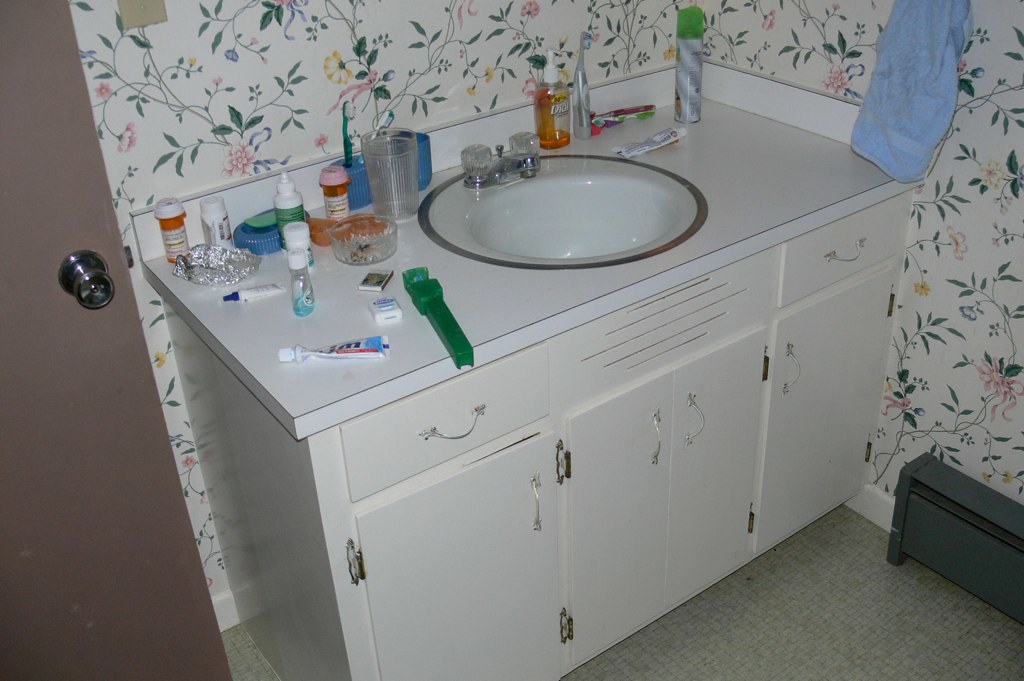The image depicts a well-used bathroom sink area set into a three-cabinet-wide vanity. Below the sink, a double-door cabinet occupies the central section, flanked by single-door cabinets on either side. Above each side cabinet, there are additional drawers, totaling two. The countertop is a pristine white surface, complemented by a modest four-inch high backsplash. 

The walls behind the vanity are adorned with wallpaper featuring a vibrant pattern of pink and yellow flowers, interspersed with green leaves and vines. Atop the countertop, a variety of personal hygiene items are scattered, including a tube of toothpaste, floss, a toothbrush, and a small travel-sized container of mouthwash. Several medication pill bottles are also present, along with a crumpled piece of aluminum foil whose purpose is unclear. 

Notably, there is a glass bowl or an ashtray, and a drinking glass, presumably for rinsing after brushing teeth. A blue copper container holding two toothbrushes is also visible, alongside a bottle of hand soap and a can of spray. An electric toothbrush and another tube of toothpaste add to the clutter. To the right side of the sink, a blue towel hangs neatly, and on the floor below, there appears to be an electric heater.